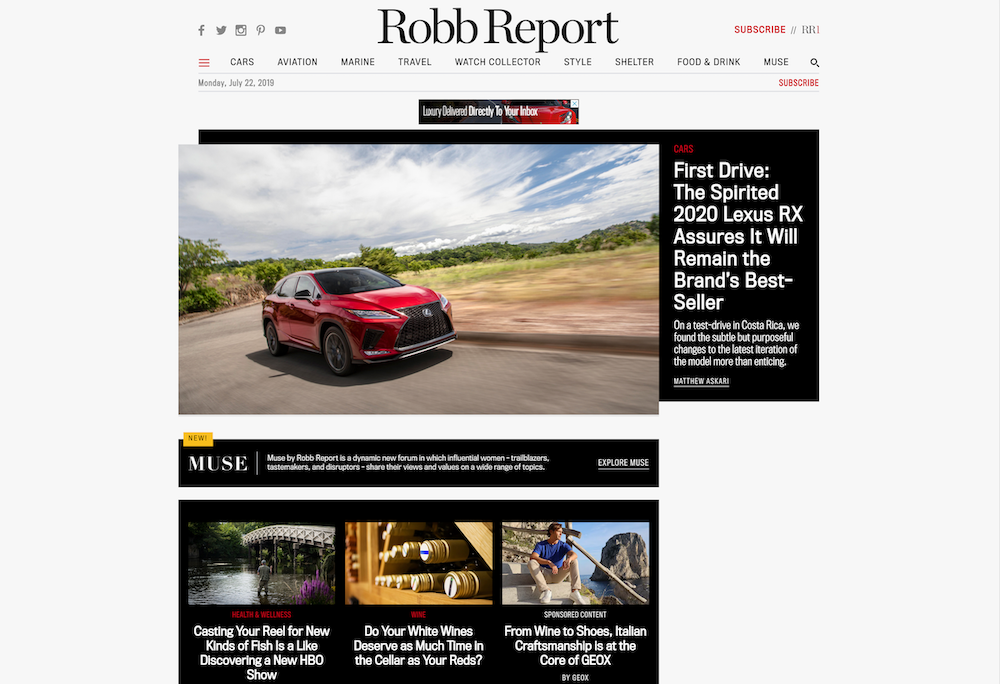The webpage is designed with a newspaper-style layout, featuring a gray background with prominent headlines accompanied by thumbnail images. At the top-left corner, social media icons for Facebook, Twitter, Instagram, Pinterest, and YouTube are positioned, likely linking to the company's respective pages on these platforms.

In bold black print at the center, the title "Robb Report" is displayed. On the top-right corner, a red "Subscribe" button with an "RR" logo is prominently placed. Below, a red menu icon with three horizontal lines provides access to various sections such as Cars, Aviation, Marine, Travel, Watch Collector, Style, Shelter, Food & Drink, and News. The date "Monday, July 22, 2019" is shown just below.

A banner with a red card stating "Luxury delivered to your inbox" is displayed under the date. An image of a red Lexus vehicle driving through a countryside highlights the leading headline: "First drive: The spirited 2020 Lexus RX assures it will remain the brand's bestseller. On a test drive in Costa Rica, we found the subtle but purposeful changes to the latest iteration of the model more than enticing," attributed to Matt Ascari.

Below this, the section titled "Muse" reads: "Muse by Robb Report is a dynamic new forum in which influential women, trailblazers, tastemakers, and disruptors share their views and values on a wide range of topics." Three additional headlines are listed beneath this section:
1. "Casting your reel for new kinds of fish is like discovering a new HBO show."
2. "Do your white wines deserve as much time in the cellar as your reds?"
3. "From wine to shoes: Italian craftsmanship is at its core at GEOX."